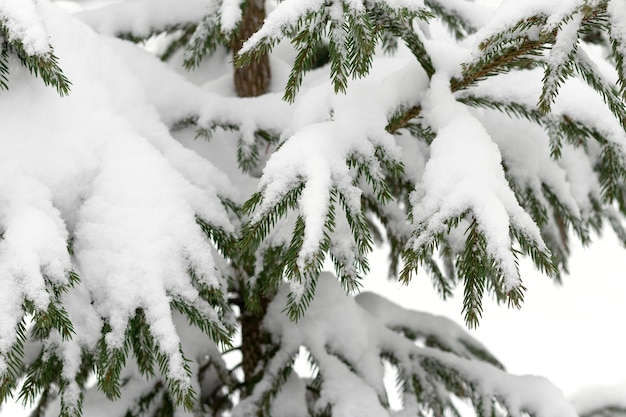This image is a very close-up, detailed photograph of a small pine tree covered in snow. The tree, likely a young evergreen, has a slim, brown trunk approximately the circumference of a human arm. Branches extend out with fern-like, needle-shaped leaves, heavily laden with powdery snow and ice. Despite the weight, the green needles can still be seen peeking through, maintaining their upright stance. The white backdrop further emphasizes the wintry and snowy setting, creating an almost surreal, isolated look as if the background either fades into a stark white snowfield or has been cropped to emphasize the tree.